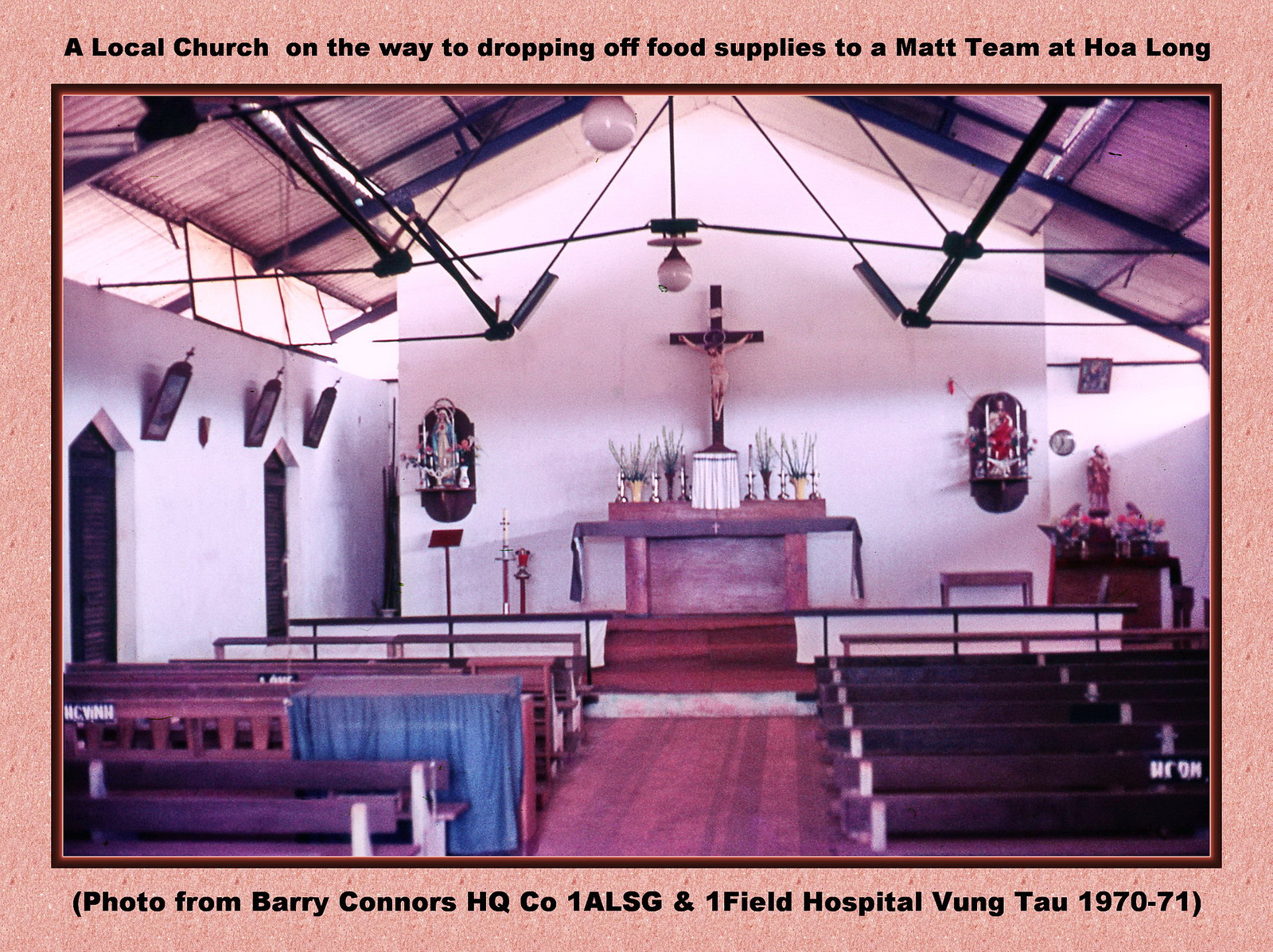The image showcases the interior of a sanctuary within an older church, distinguished by wooden floors and rows of wooden pews facing the front. Central to the scene is a large crucifix with a depiction of Jesus affixed to a white wall. The altar below the crucifix is adorned with various religious artifacts, including candles and possibly plants. The space is further accentuated by hanging lights from the ceiling and additional decorations such as statues, flower arrangements, and paintings along the walls. There's a notable absence of people, giving the scene a serene, postcard-like quality. A specific pew displays a white and blue curtain or sheet. A pinkish salmon-colored border surrounds the image, with black text at the top stating, "A local church on the way to dropping off food supplies to a MAT team at Hoa Long." The bottom text reads, "Photo from Barry Connors, HQ Co. 1 ALSG and 1 Field Hospital, Vung Tau, 1970-71," indicating the historical context of the photograph. The overall color scheme of the interior includes hues of peach, pink, blue, and white.